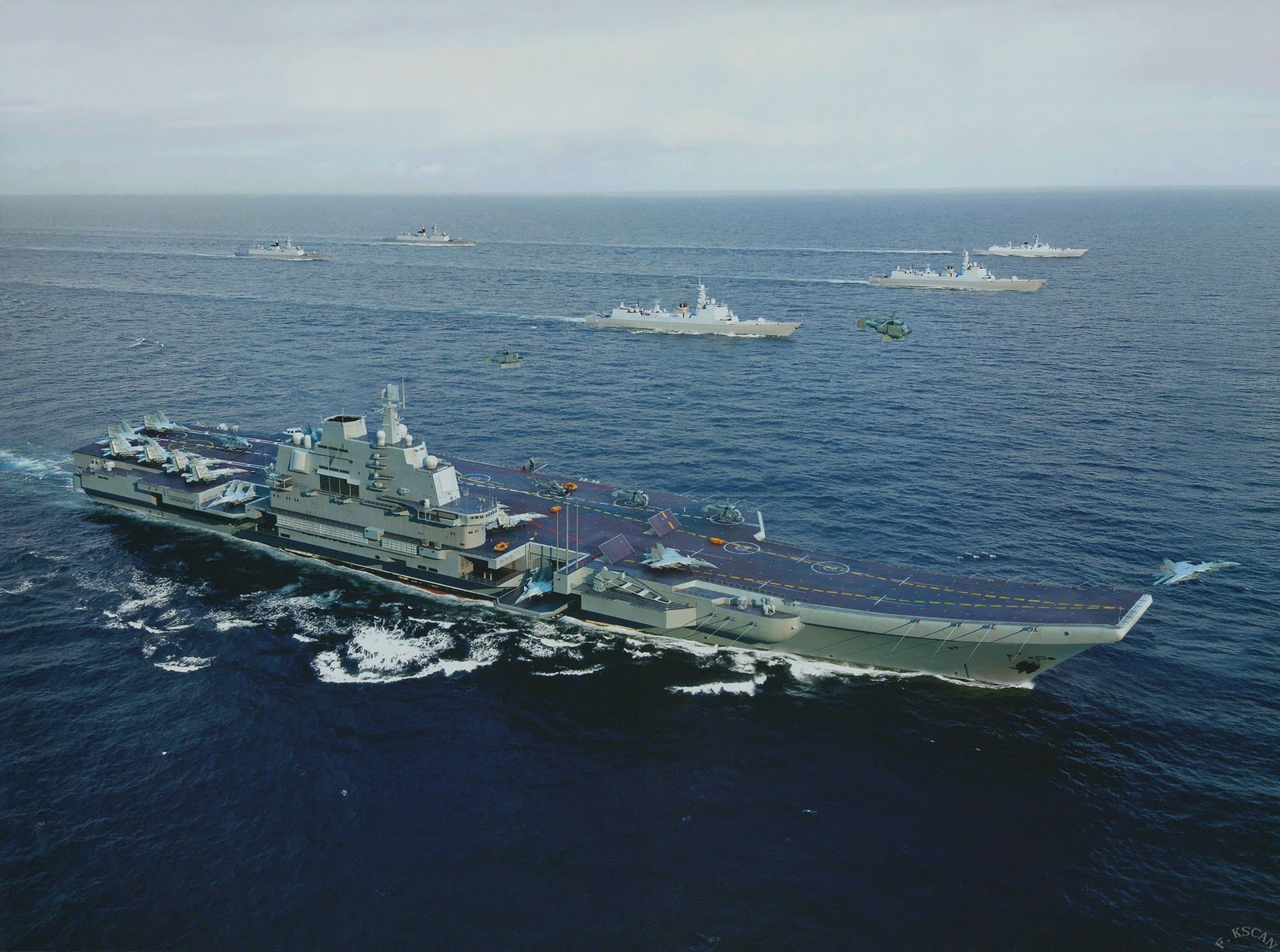The photograph captures a vast ocean scene, where deep blue waters blend with a light blue, slightly cloudy sky. Dominating the foreground is a large aircraft carrier, featuring a runway with a yellow line and several aircraft parked on its deck. Notably, one aircraft is taking off from the very tip of the carrier's runway. To the left side of the carrier, there are multiple jets and at least three helicopters stationed. Surrounding the aircraft carrier are five escorting warships, likely destroyers or frigates, positioned at varying distances but maintaining a cohesive formation as they travel together. In the midst of this naval convoy, a helicopter hovers above the water, adding to the dynamic nature of the scene. The image exudes a military feel with its impressive display of naval power and coordination under a slightly overcast yet serene sky.